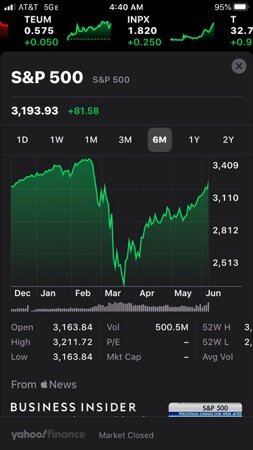This image is a detailed screenshot of a mobile phone displaying a stock market application. At the very top of the screen, the status bar indicates three bars of service, an 'AT&T 5G' network, the time '4:40 AM,' and a battery icon showing 95% charge. Below the status bar is a moving banner with various stocks and their daily gains.

The main focus of the screenshot is the S&P 500 section, showcased on a sleek black background with a slightly lighter black for emphasis. The S&P 500 index is listed at '3193.93,' displaying a positive change of '+81.58' in vibrant green text. A graphical representation of the index is provided below, featuring a green shaded bar graph. The graph is set to the six-month view, with important value amounts marked on the right side and months of the year labeled along the bottom.

Further below, detailed stock data is split into categories including 'Open,' 'High,' 'Low,' 'Volume (VOL),' 'P/E ratio,' and 'Market Cap,' each populated with specific numeric data. At the very bottom, the screenshot credits a source: "Apple News" and "Business Insider" in prominent white text.